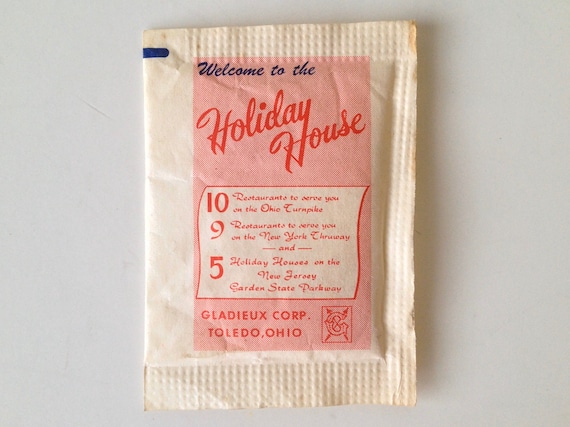This image displays a vintage sugar packet from a restaurant or hotel named Holiday House, set against a white background. The packet itself is a small, vertical rectangle with a cream-colored base and a slightly worn appearance, featuring some browning at the edges. It prominently showcases a navy blue script at the top that reads "Welcome to the" followed by "Holiday House" in red, angled cursive. Below that, bold red numbers highlight the locations of the Holiday House chain: "10 restaurants to serve you on the Ohio Turnpike," "9 restaurants to serve you on the New York Thruway," and "5 holiday houses on the New Jersey Garden State Parkway." The packet is marked with "Gladue Corp., Toledo, Ohio" at the bottom, indicating its manufacturer. The detailed and slightly aged design adds a touch of nostalgia to this sugar packet, often typical of those found in hotels or resorts to be torn open and used in beverages like coffee.